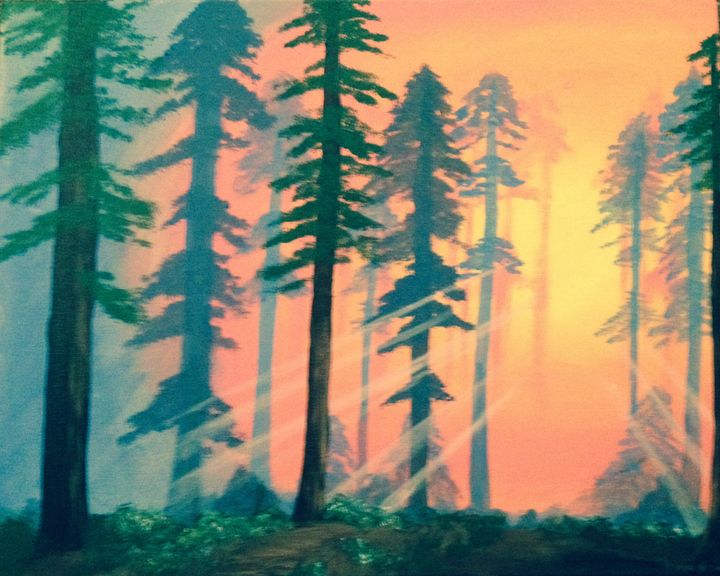This image depicts a vibrant, artistic interpretation of a forest at either sunrise or sunset. Dominated by towering, slender trees with dark brown trunks and lush green leaves, the foreground showcases a dense, flourishing forest. Smaller bushes pepper the ground, contributing to the rich greenery. A narrow dirt trail meanders through this serene woodland setting.

In stark contrast, the backdrop explodes with color, featuring a brilliant sun that radiates intense yellow rays, seamlessly blending into an orange and red sky. This radiant hue engulfs the right side of the image and gradually transitions into green toward the left. The sun's powerful illumination is so striking that it evokes the impression of an explosive force, though no smoke is present. Despite some suggestions of a forest fire or smoky atmosphere due to the blurry, low-quality nature of the image, the scene most likely captures the ethereal beauty of a sunrise or sunset filtering through a foggy or mist-laden forest.